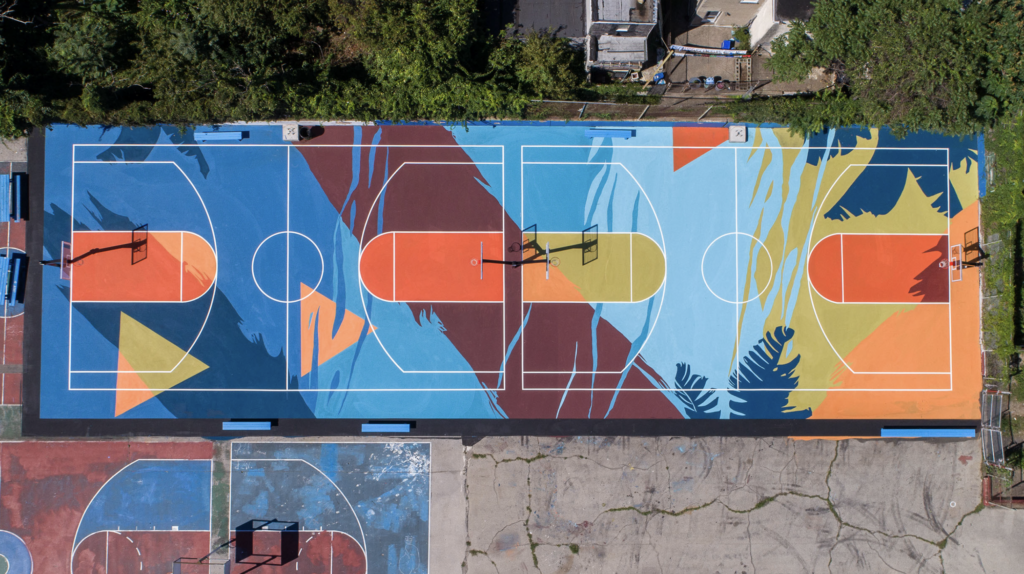This aerial photo, taken from approximately 50 feet above, captures a vibrant and artistic basketball court with two courts side by side. The court features a striking abstract design, predominantly using colors such as brown, olive green, blue, and orange. The intricate layout includes the clearly visible white lines denoting the three-point shot areas, free throw lanes with their missile-shaped setups, and central circles of each court. The left court showcases a transition from darker to medium and light sky blue tones, with an artistic stripe of dark blue and geometric shapes like gold and orange triangles and a maroon stripe intersecting the courts. The right court features a gold and orange palette with a vivid blue palm tree outlined near one part. Poles for the basketball hoops are evident, though the hoops themselves are not visible. Beyond the courts, the top of the image displays the tops of trees and parts of buildings in the upper right corner. In the bottom left, there appears to be another athletic court of indeterminate sport, and more concrete is seen toward the bottom of the image.